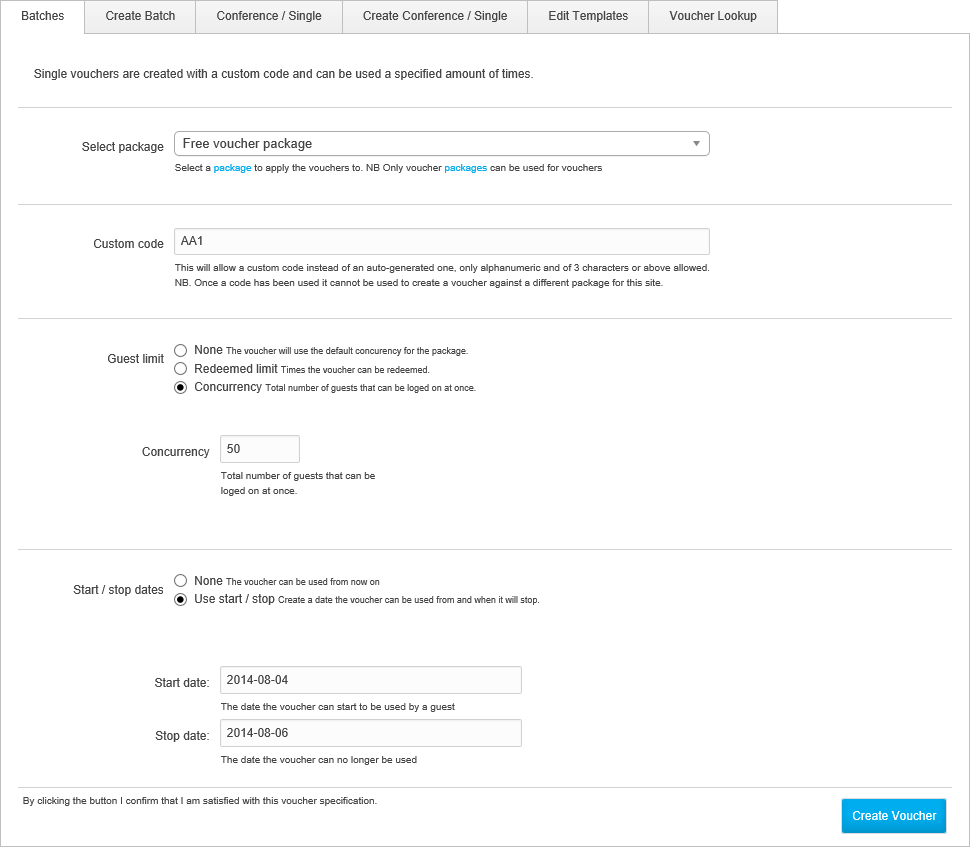This image displays a web page designed for managing and creating vouchers. At the top of the page, there are several navigation categories: Batches, Create Batch, Conference/Single, Create Conference/Single, Edit Templates, and Voucher Lookup.

Lower on the page, a section explains that single vouchers are created with a custom code and can be used a specified number of times. Under the "Select Package" submenu, there is an option for a Free Voucher Package with a drop-down box indicating, "Select a package to apply the vouchers to," noting that only specific packages can be used for vouchers.

A box labeled "Custom Code" shows an entered value of "AA1." A note specifies that this allows for a custom code instead of an auto-generated one, with the requirement that codes must be alphanumeric and at least three characters long. Additionally, once a code has been utilized, it cannot be reused for creating vouchers under a different package for this site.

Under "Guest Limit," three options are provided: 
1. None – The voucher uses the default concurrency for the package.
2. Redeemed Limit – Indicates the number of times the voucher can be redeemed.
3. Concurrency – Specifies the total number of guests that can be logged on at once. The Concurrency option is currently selected, with a field below indicating a limit of 50 guests.

Further down, the "Start-Stop Date" feature is described, allowing for the creation of a date range during which the voucher is valid. The Start Date is set to 2014-08-04, and the Stop Date is 2014-08-06.

At the bottom of the page, a confirmation message reads, "By clicking the button, I confirm I am satisfied with the voucher's specification," followed by a prominent blue "Create Voucher" button.